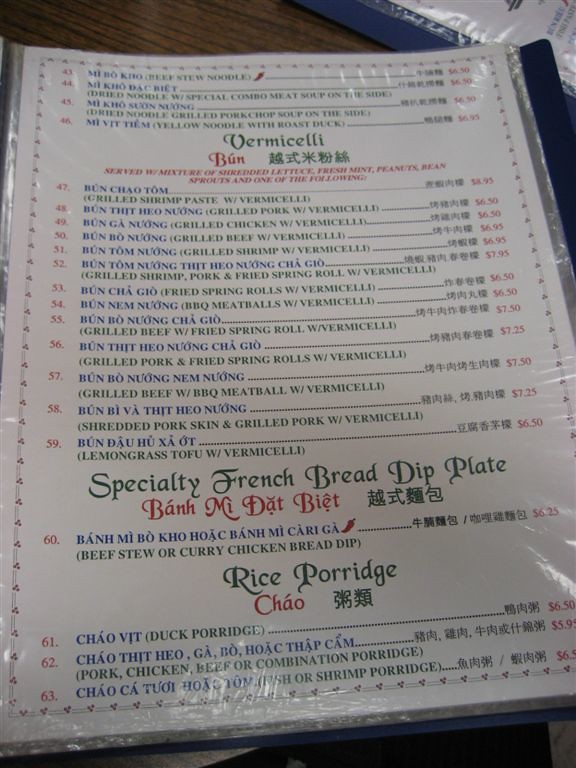A slightly angled menu, encased in a transparent plastic cover that exceeds its size, lies on a wooden surface. The majority of the image is occupied by the menu itself, set at an estimated 5-degree tilt to the left. The menu features a white background with items listed and organized neatly. Each item number is printed in red on the left, while the corresponding price is in red on the right. The names of the dishes appear in blue, accompanied by descriptions in dark green.

At the top, the first section contains five items numbered 40, 3, 4, 5, and 6, respectively. Below this, in large green print, the word "Vermicelli" stands out. The section also includes some text in red and additional green characters, contributing to the menu's multilingual presentation. Following this, two red lines separate a list of items numbered 47 to 59.

A prominent green heading reads "Specialty French Bread Dip Plate," followed by another red line and green text. Item number 60 occupies the space beneath it, succeeded by "Rice Porridge" in bold letters. Further down, red words and green characters introduce items numbered 61, 62, and 63. 

The menu is framed by a subtle yet slightly decorative outline, providing a gentle border that encapsulates the detailed information within.